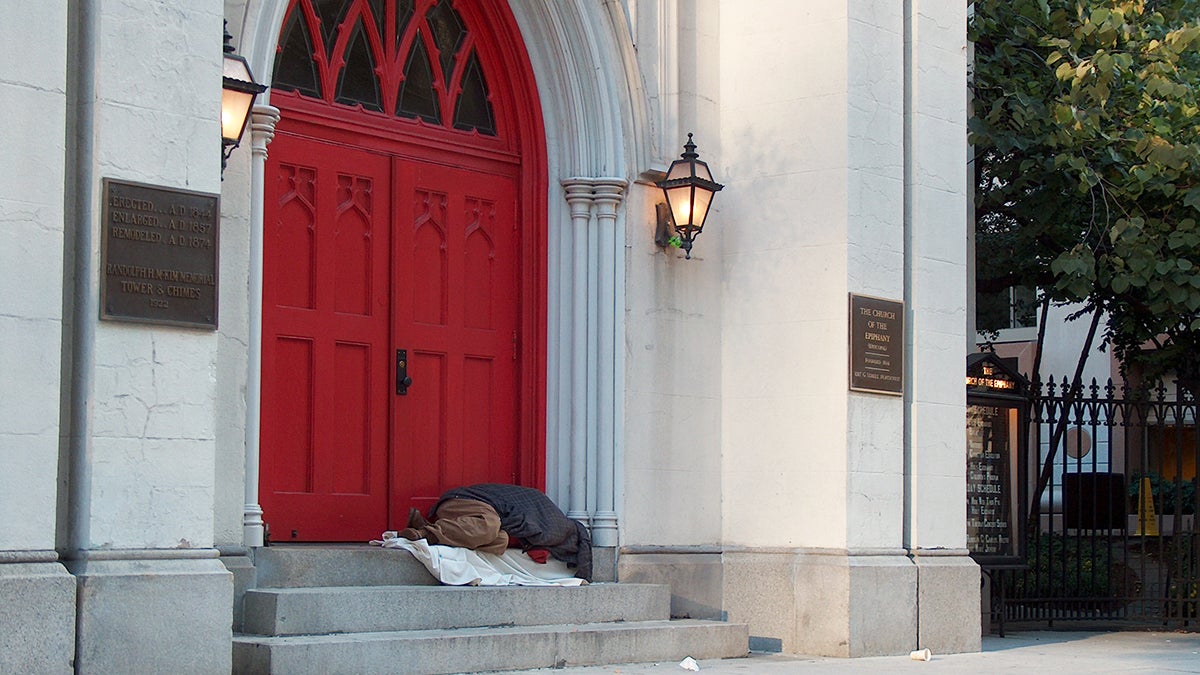This color photograph, captured in landscape orientation, showcases the front facade of a city street church. Dominating the left side of the image, the church's iconic red double doors stand out, set within an arched entryway flanked by ornate lantern-style light fixtures. Bronze plaques, although the inscriptions are illegible, are mounted on either side of the entrance, adding to the historical character of the building. 

Three concrete steps lead up to these doors, and on the topmost step rests a person, shrouded in a white blanket, seemingly asleep. The individual wears a light-colored cap or has light hair, and dons a dark jacket, though their facial features are not visible. 

Adjacent to the church on the right, black wrought iron fencing encloses a small area, while a brightly lit reader board displays the church's schedule of events, adding a touch of modernity. A dark tree looms in the top right corner, framing the scene with natural elements. The overall photographic style leans towards representational realism, capturing the details and atmosphere of this urban religious sanctuary.